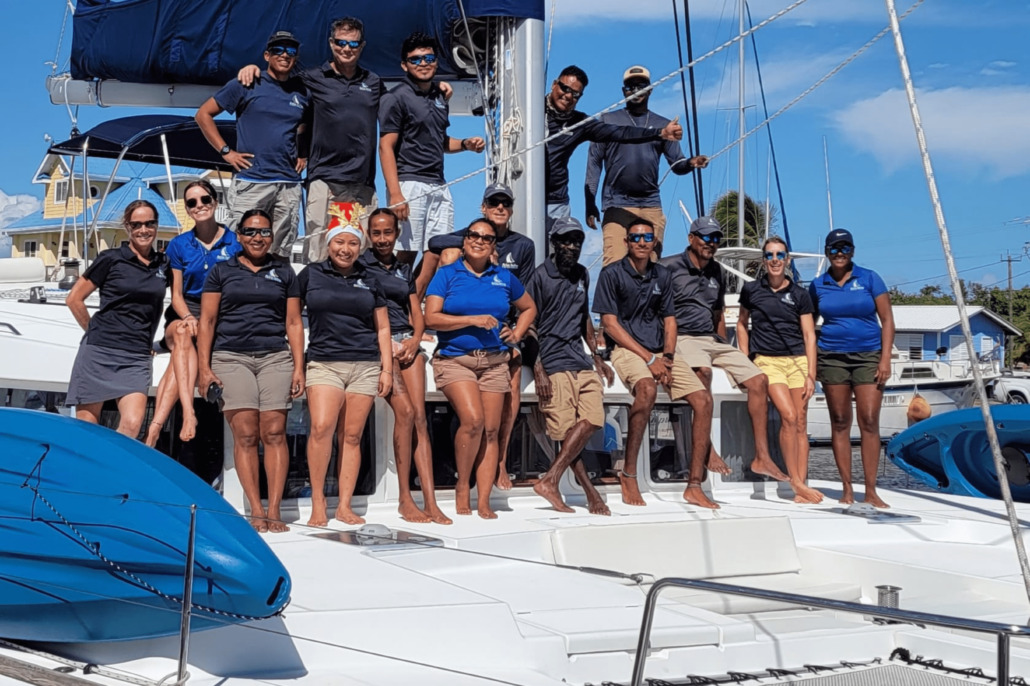This landscape photograph captures a diverse and cheerful crew of about 10-15 individuals standing on the front deck of a large white sailboat. The boat is flanked by blue kayaks on both sides, and a clear blue sky serves as the picturesque backdrop. The crew members are a mix of men and women, wearing short-sleeved collared shirts in shades of navy, bright blue, and black, paired with khaki, gray, or yellow shorts and skirts. The central rows show most individuals standing, with a couple seated on raised parts of the deck, while the back row stands elevated, some with arms around each other. Many wear sunglasses and some have hats, adding to the relaxed, sunny-day vibe. They all wear matching shirts featuring an indistinct logo, and everyone is smiling warmly into the camera, exuding happiness and camaraderie.